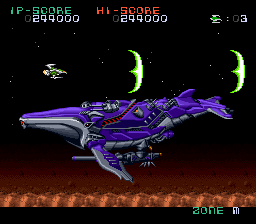In this detailed image from the video game Gradius, the top left corner displays the player’s score as "1P-SCORE 0299000," mirroring the high score shown at the top. Below the scores, the interface indicates "BASE-TO-BASE SHIP CALLING 03." Prominently featured in the center is a distinctive green ship, emitting green energy blades. Towering over the scene is an intricately designed blue whale. Its underside is silver, and it sports a red stripe along its middle, contrasting against its vivid blue body. The whale appears to be covered in patches of brown fur, giving it a unique, almost mythical appearance. Near the bottom right, "ZONE M" is denoted within a black rectangle, providing a sense of location within the game. The background is diverse, with brown hues transitioning into black at the top, suggesting a deep-space or cosmic environment. Various other sci-fi-themed whales can be seen populating the scene, adding to the fantastical and otherworldly atmosphere.